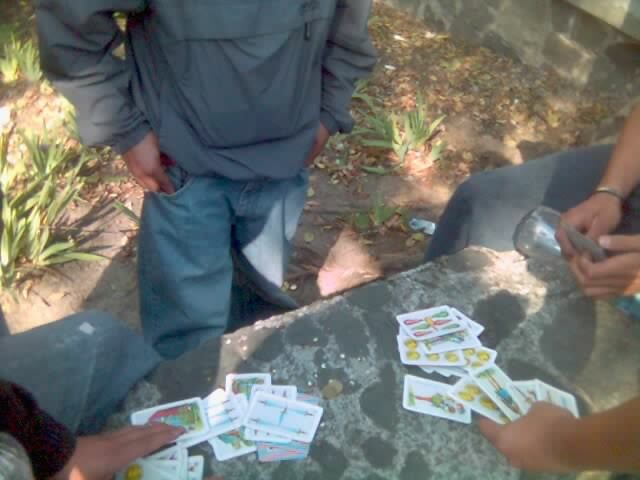In the image, three individuals are engaged in a card game, positioned around what appears to be a stone bench held together by mortar or concrete. The scene captures one person standing and two seated. Their game involves distinctive cards, many of which are laid out face up. Notably, there are cards displaying varied symbols such as five swords arranged in an 'H' pattern, three swords on another card, several cards featuring people, and cards with round, unclear symbols. One card showcases multicolored droplets arranged in numerical patterns, which could be something like a "seven of carats or drops." This assortment strongly suggests they may be using tarot cards, given the evocative imagery of numbered swords and illustrated figures.

The most visible participant is dressed in a gray pullover coat with long sleeves, a front zipper pocket, and blue jeans. On the left, another person is identifiable by their gray pants and a copper bracelet adorning their right hand. From the lower right corner of the scene, a hand extends into the frame, holding a few cards. In the lower left corner, a partial view of another individual shows a leg and a hand clad in a black sleeve, also likely wearing blue jeans. The background features a garden area with sparse, somewhat scruffy plants, adding to the rustic ambiance of the setting.